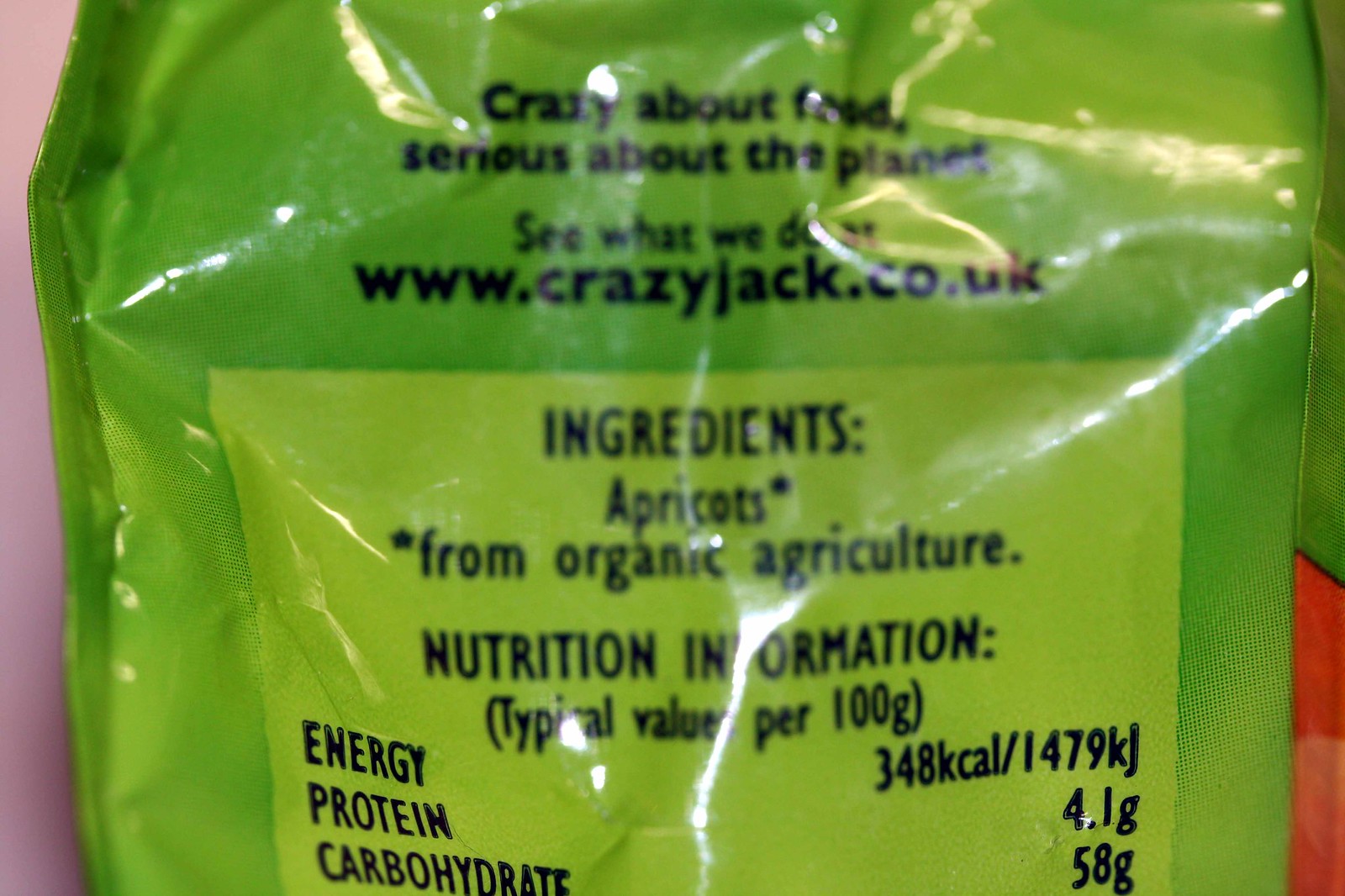The photograph showcases the back of a bright green plastic food package with two distinct shades of green. Dominating the top of the package, bold black text reads, "Crazy about food, serious about the planet," followed by a prompt to "See what we do at www.crazyjack.co.uk." Below this, a lighter green square highlights the ingredients section, stating "Ingredients: Apricots*" with an asterisk indicating the apricots are from organic agriculture. The nutritional information is detailed in black font, listing typical values per 100 grams: Energy 348 kcal / 1479 kJ, Protein 4.1 g, and Carbohydrates 58 g. This packaging reflects the company’s commitment to organic food and environmental sustainability.